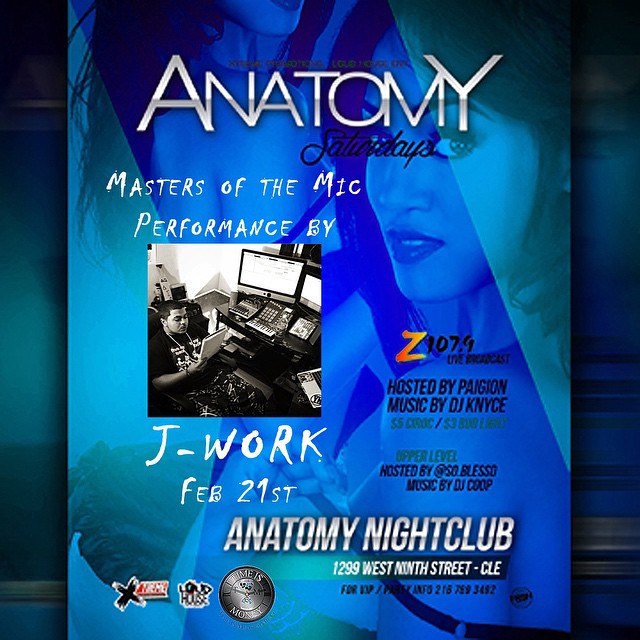The advertising poster features an intricate, blue-themed design with two women in the background. One woman's face is seen sideways, while the other is visible from the neck down, creating a prism-like visual effect in blue and green hues. At the top of the poster, bold white letters spell out "ANATOMY," with "Saturdays" elegantly written below in black cursive. Beneath this, in white font, it announces "Masters of the Mic," followed by "Performance by J-Work." 

The central image is a black and white photo of a man at a computer, perhaps a DJ, holding a piece of paper or notebook and adorned with a gold necklace. Details include the performance date, February 21st, and the event location at Anatomy Nightclub, 1299 West 9th Street, Cleveland. 

To the right, Z107.9 Live Broadcast is highlighted, with the evening hosted by Pagan and music by DJ Nice. More event details promote Ciroc for $5 and Bud Light for $3 on the upper level. The event is also hosted by "So Bless," with additional music by DJ Corp. The nightclub's contact information is provided at the bottom for further details.